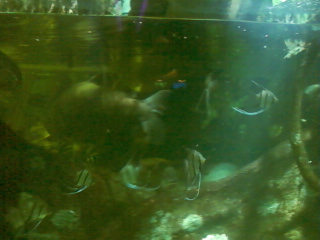In this small, square, low-resolution photograph of a murky fish tank, the water has a green tint that diminishes visibility, casting a hazy glow over the scene. The lighting is poor, adding to the overall pixelated and blurry quality of the image. In the center and near the bottom left of the tank, you can see around four or five fish distinctly while hints of a couple more are also visible. The fish include angelfish, distinguishable by their black dorsal fins, red and black stripes, yellow bodies, and long, wing-like fins. There is also a large carp, evident from its brown tail, and some smaller blue and orange fish scattered around. The tank’s bottom is adorned with rocks, especially a prominent light brown one on the right, tinted green by the water. Additionally, there are patches of vegetation spread throughout the tank. At the very left, the glass’s reflection partially captures a man wearing a black shirt with dark hair. A light source from above highlights parts of the sand and rocks at the tank's bottom, adding a final touch to this indoor aquarium display.